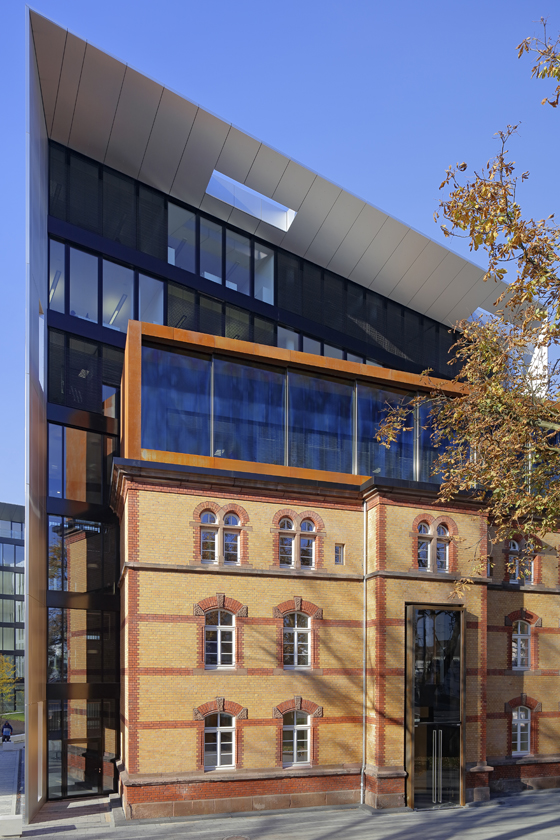The image showcases the facade of an architecturally complex and modern building, consisting of two distinct sections. The front section has an orange wall highlighted with tan and brighter orange accents, featuring a total of ten square windows arranged in three visible rows: four in the top row, three in the middle, and three at the bottom. This section also has a large, black, two-floor tall entryway at its center. The topmost part of this front section boasts a large see-through window wall with dark blue, reflective windows. Adjacent to this is a taller, more modern structure that looms above the orange facade, characterized by its seven floors of reflective mirror windows. Some windows on the top floor have dark black curtains, making them less reflective. Additionally, a small segment of the wall protrudes on the upper right side. A cement walkway also leads up to the entry, bordered by a small tree, complementing the contemporary style of the building.